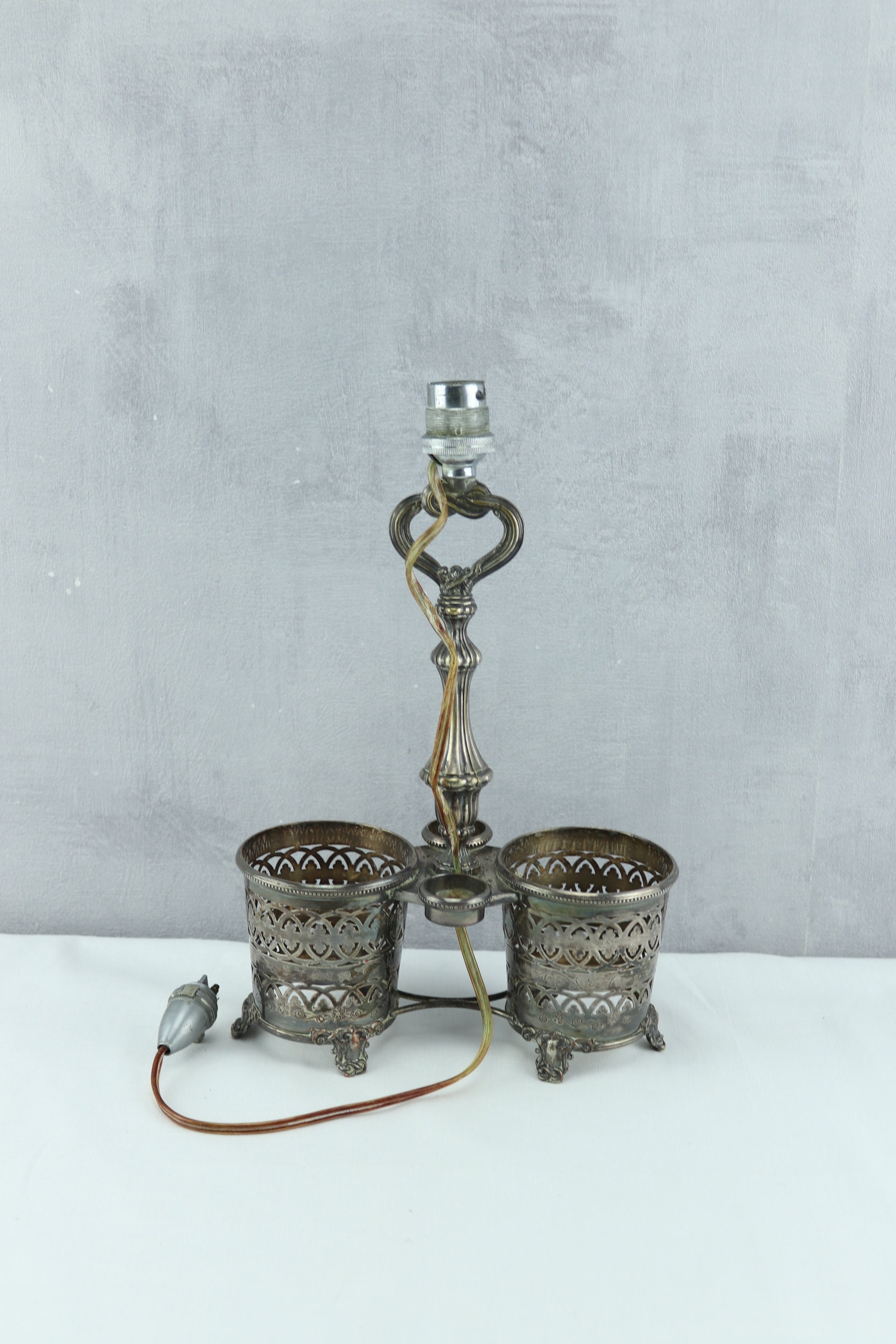This photograph depicts a vintage silver lamp, highly tarnished, set against a light gray background on a white tabletop. The lamp is devoid of a light bulb and lampshade, revealing a socket at the top for screwing in a bulb. A short cord emerges from this socket, leading to an old-fashioned, bulky plug. The lamp features an intricate design: an oblong loop descends from the top, joining a flared silver stem that connects two ornately etched cylindrical metal baskets. These baskets rest on decorated feet, suggesting an additional function possibly for holding candles. The entire piece, with its filigree pattern and elaborate craftsmanship, reflects a bygone era, blending utility with antique charm.